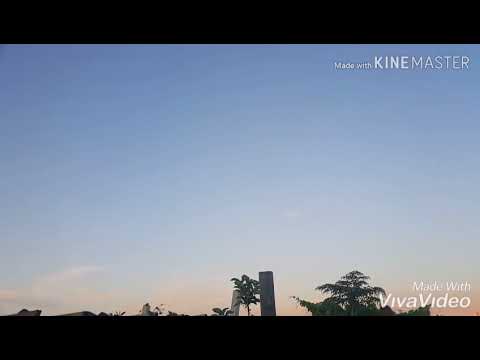The image is a scenic photograph bordered by black bars at the top and bottom, creating a slide-like appearance. The centerpiece is a stunning sky that transitions from a dark blue at the top to a pale pink, almost peach, at the horizon, reminiscent of a serene dusk setting. Wispy white clouds float on the horizon, complemented by silhouetted trees, a shrub, and the cropped tops of a few buildings peeking into the frame. The scene includes two distant skyscrapers, adding a touch of urbanity to the otherwise natural landscape. The upper right corner of the image is marked with the white text "Made with KineMaster," while the lower right corner bears the similar inscription "Made with Viva Video," indicating some element of digital manipulation or video editing.